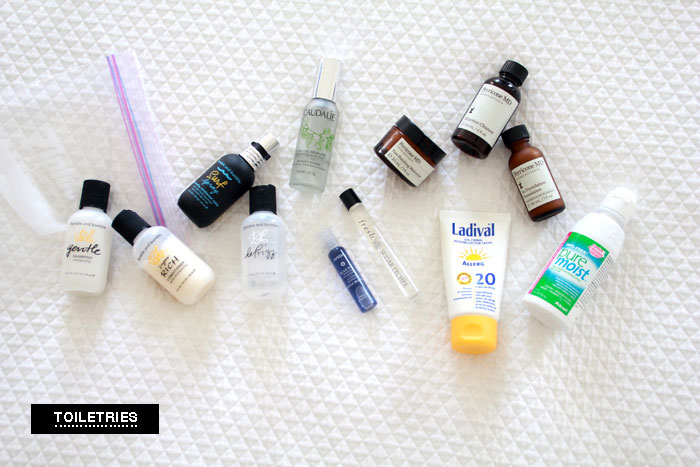The image features an array of toiletries arranged in an organized manner. 

In the bottom left corner, the word “toiletries” is displayed in white text. Positioned next to this text is a white bottle with a black cap. To the middle left, there is another white lotion bottle, also with a black cap. Adjacent to these, a third bottle has a black cap with a silver top, and right beside it is a clear liquid bottle with a black cap.

A little further to the right is a white bottle capped with a silver metal lid. There's another white bottle topped with a yellow cap. On the far right, there is a "Pure Moist" bottle featuring a green label.

Additionally, the lineup includes a brown bottle and a black bottle, both equipped with black caps. In the center, there are two mini bottles: a blue one and a clear white one, each with a black cap. 

The assortment displays a variety of packaging and cap styles, suggesting different types of products within the toiletries category.